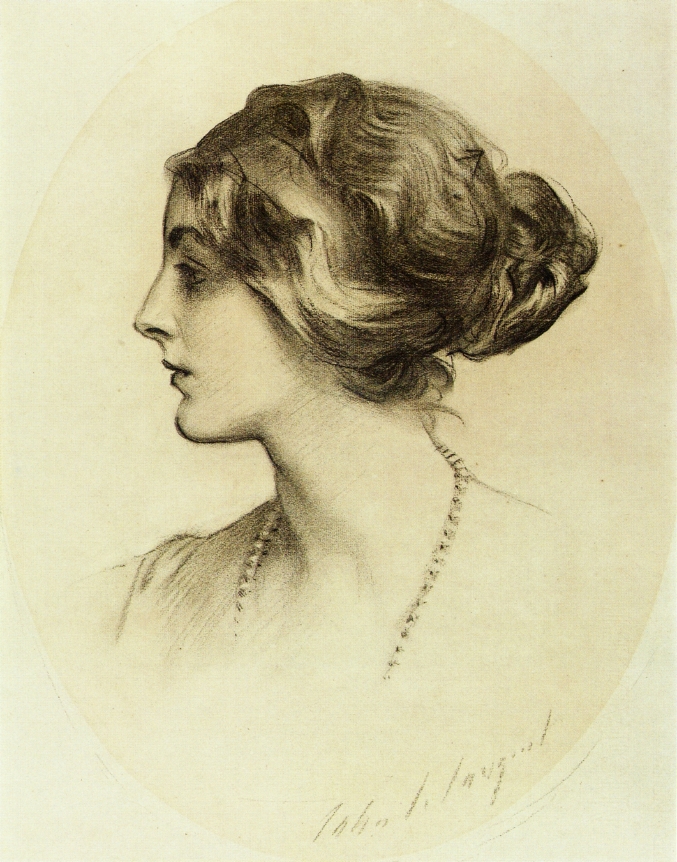This is a detailed sketch of a woman in profile, drawn against a faded yellow background. She is looking thoughtfully to her right, showcasing her delicate and elegant features. Her hair, likely brown, is styled in a wavy, yet slightly messy bun at the back of her head. The simplicity of her look is complemented by a long necklace, possibly pearls, which adds to her poised appearance. The sketch, meticulously shaded with fine lines, captures only her head, neck, and a hint of her shoulders and dress, devoid of other ornamentations. The artist, whose full name—possibly John Langood—is partially signed at the bottom right of the sketch, highlights her fair, light skin and classic, refined beauty. The image’s minimalist style and muted tones suggest it might have been created for an advertisement or a portrait study.